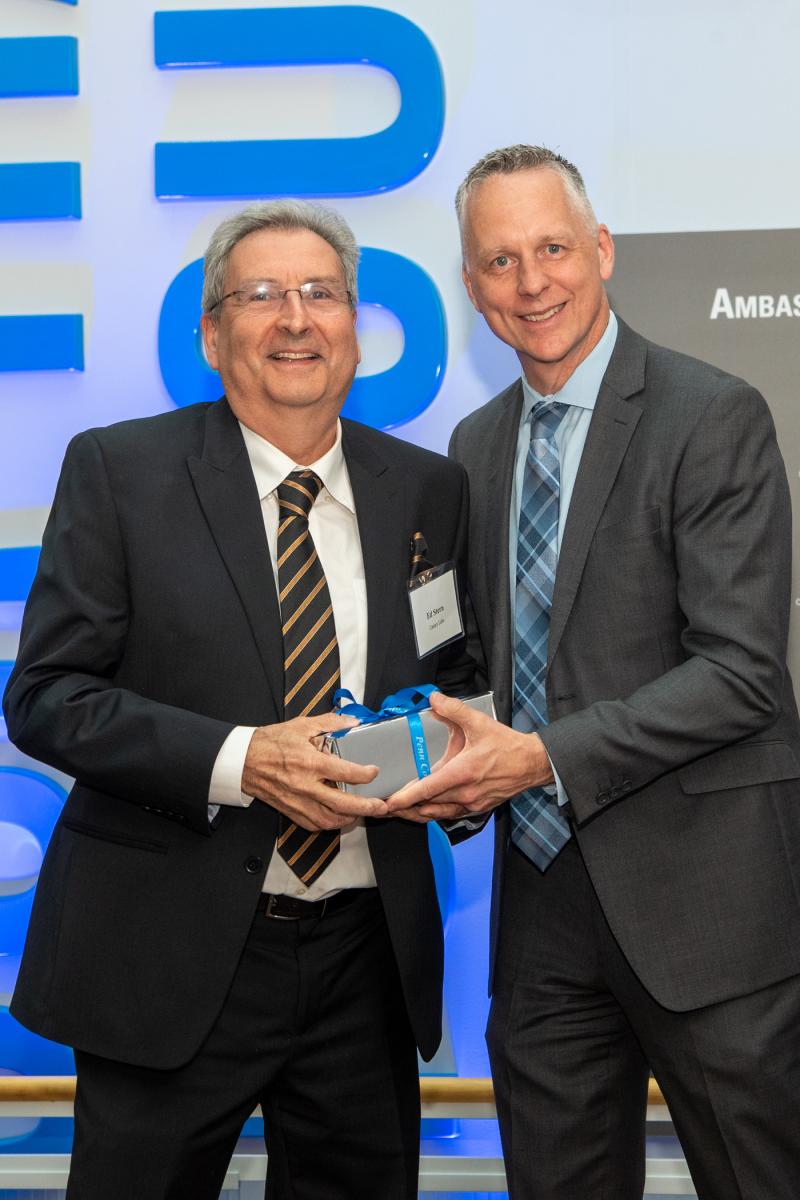In the image, two Caucasian men, who appear to be businessmen, stand side by side and smile warmly for the camera. Both are holding a small, silver-wrapped present adorned with a bright blue bow, each having one hand on the gift. The man on the left, an elderly gentleman with white hair and glasses, sports a big smile and is dressed in a black suit comprising a black sport coat, black pants, a black belt, a white shirt, and a black tie with gold stripes. He also wears a name tag in a clear plastic holder attached to his suit. The man on the right is taller and slimmer, possibly in his 60s, with cropped silver-gray hair and no glasses. He is dressed in a deep gray suit, a light blue shirt, and a three-toned blue plaid tie. The background they stand against is primarily blue, featuring partial words and deep blue letters, one of which appears to spell "ambassador". The rest of the text is indistinct.